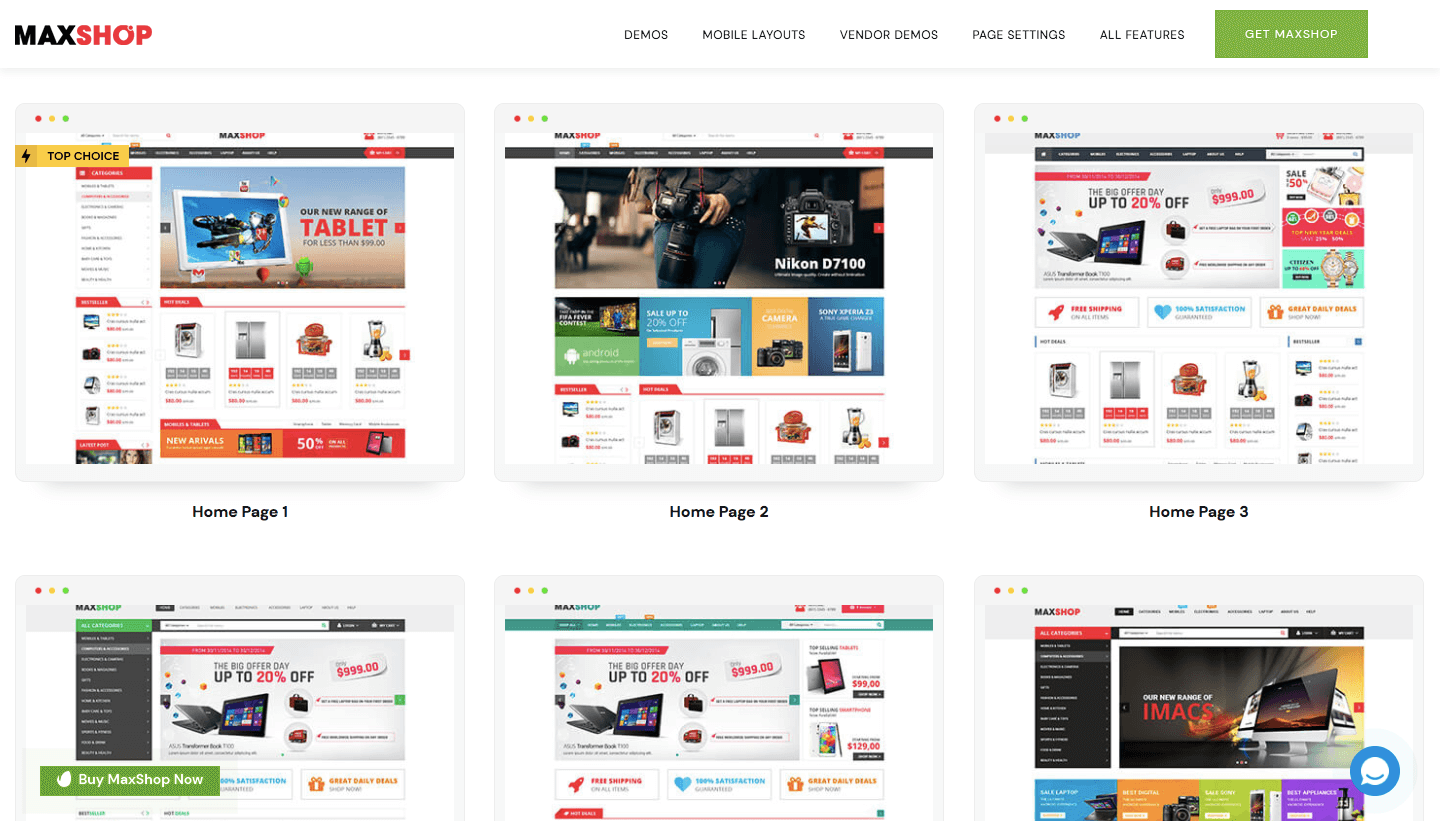This screenshot captures the homepage of an online store specializing in website templates. The website features a clean, predominantly white background. At the top, there is a white navigation bar where the site’s name is displayed: "max" in black font followed by "shop" in red font. 

To the right of the site name, there are several clickable options: "Demos," "Mobile Layouts," "Vendor Demos," "Page Settings," and "All Features." Below this navigation bar, the main page showcases six different homepage layout options, organized in two rows of three. Each layout option is clearly labeled as "Homepage One," "Homepage Two," and "Homepage Three"; however, the labels for the layouts in the second row are cut off.

In the lower right corner of the screen, there is a blue chat bubble icon, likely a link to a chatbot service intended to assist visitors with their shopping experience. This detail underlines the website's customer service feature.

Overall, the website specializes in selling templates for websites, providing users with multiple layout options that, while somewhat similar in appearance, offer various starting points for design customization.